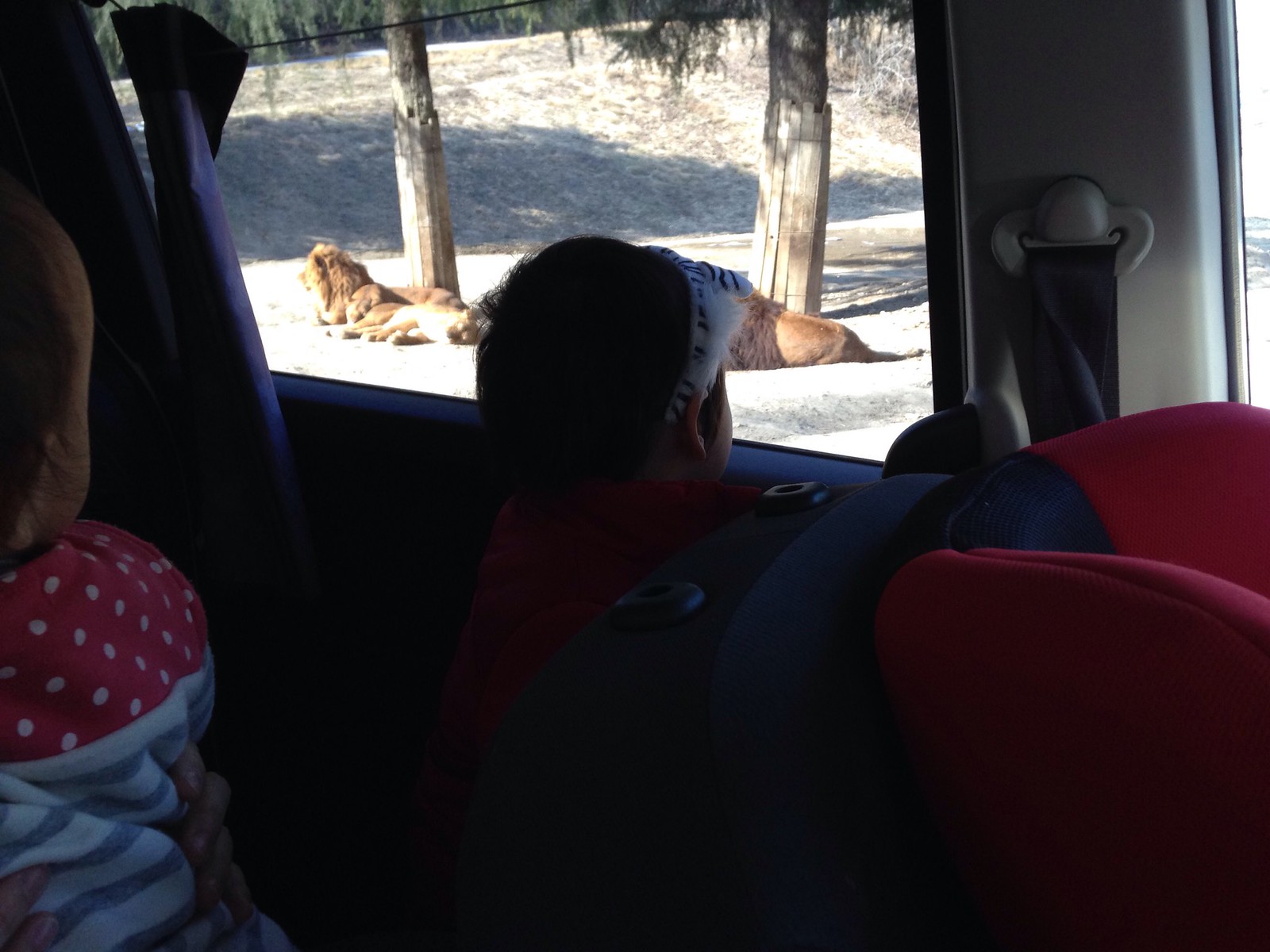A detailed photograph captures the scene from inside a car, likely during a drive-thru safari or zoo. The interior, viewed from the passenger side, shows two young children: a boy approximately five or six years old wearing a toy cap, and a baby in a car seat. The baby wears a red and white polka dot shirt with blue stripes. The car features red seats, one of which might be a baby's car seat. Through the window, two male lions with full manes are lounging on what appears to be a concrete surface. The lions are sunbathing near two tree trunks, which provide little to no shade. The ground outside is either concrete or a very gray grass, surrounded by some green leaves from the trees.